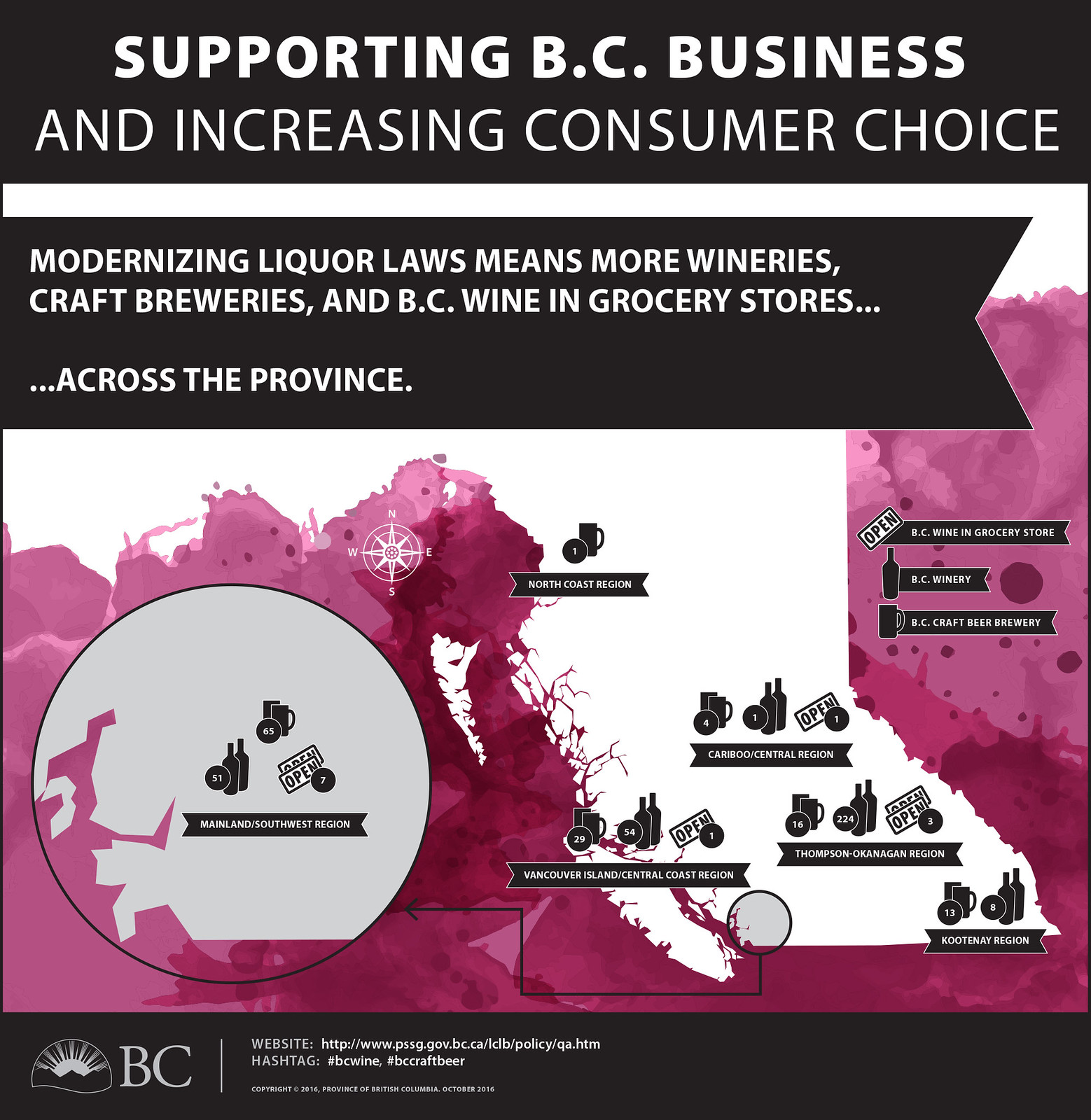This image is a detailed infographic from October 2016 related to the province of British Columbia. It emphasizes supporting BC business and increasing consumer choice through the modernization of liquor laws. The graphic features a black border with a horizontal band and centered text in white that reads "Supporting BC Business and Increasing Consumer Choice." Below this is a black ribbon containing text that states, "Modernizing liquor laws means more wineries, craft breweries, and BC wine in grocery stores across the province." The graphic highlights numerous regions within British Columbia affected by these changes, including the North Coast Region, and is accented with images of wine bottles and cups. It also incorporates a mix of black and white with a central portion in purple coloring. Hashtags associated with the infographic include #BCWine and #BCCraftBeer. Additional information is available at www.pssg.gov.bc.ca.klv.policy.qa.htm.